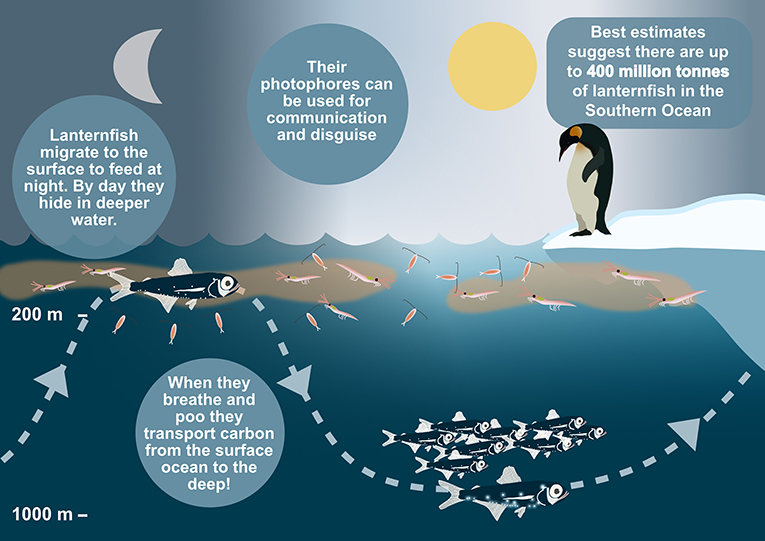This illustrated infographic depicts the life cycle and behaviors of lanternfish in a detailed, cartoonish style. It features a grey sky with a sun at the top center and a crescent moon at the top left. A penguin stands on a small ice piece on the right, gazing into the blue, splotchy-brown water below. The infographic includes several informational word bubbles connected by dotted arrow lines, explaining key points about lanternfish. 

The first bubble states, "Lanternfish migrate to the surface to feed at night. By day, they hide in deeper water," with arrows showing their movement from 1,000 meters deep to around 200 meters. Another bubble explains, "When they breathe and poo, they transport carbon from the surface ocean to the deep." A third bubble mentions, "Their photophores can be used for communication and disguise." Finally, a bubble at the top right notes, "Best estimates suggest there are up to 400 million tons of lanternfish in the southern ocean." Elevation markings on the left further illustrate the depths mentioned, and additional visual elements such as shrimp and schools of lanternfish provide context to their feeding habits and population density.